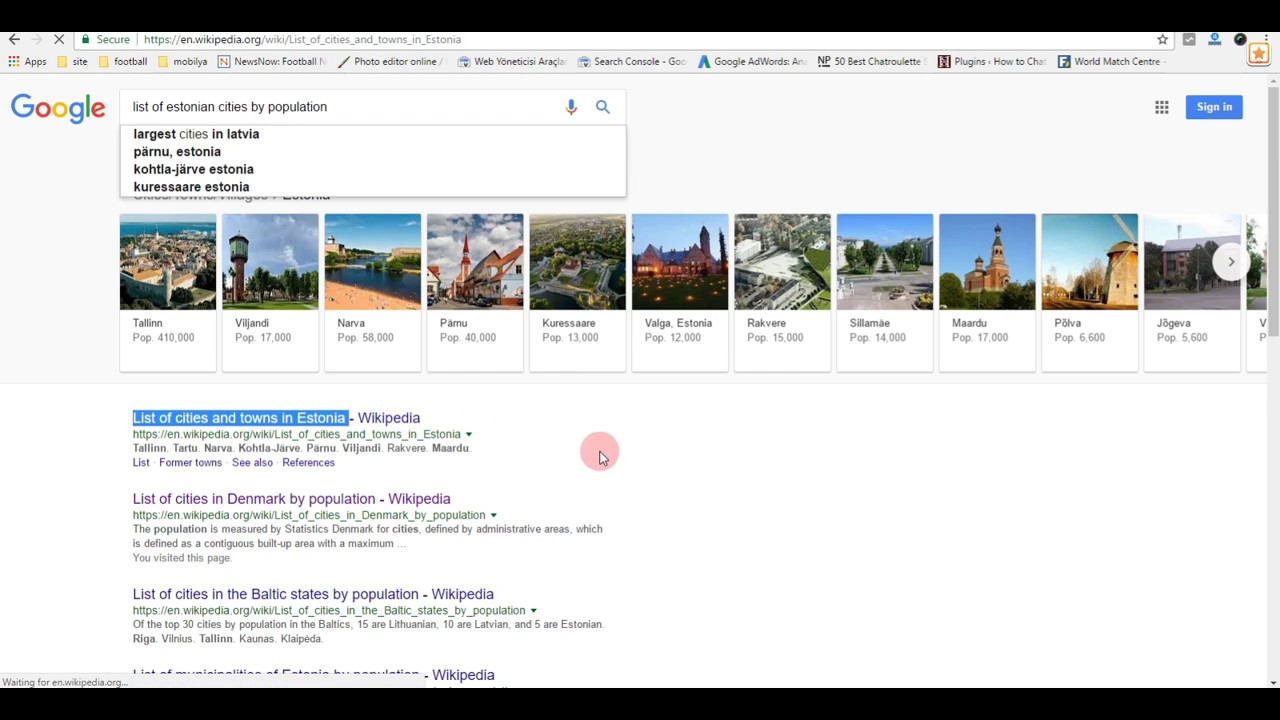The image shows a Google search result leading to Wikipedia. At the top of the page, the domain wikipedia.org is visible. The search query is "list of Estonian cities by population," accompanied by several images of cities and their respective populations. Notable cities listed include:

- Tallinn with a population of 410,000
- Pajandi with 17,000
- Narva with 58,000
- Pamu with 40,000
- Kursar with 13,000
- Volga, Estonia with 12,000
- Rakver with 15,000
- Silamay with 14,000
- Mardu with 17,000
- Polva with 6,600
- Jojeva with 5,600

Below these summaries, there is a list of clickable Wikipedia articles related to the search, such as "List of cities and towns in Estonia," "List of cities in Denmark by population," and "List of cities in Baltic states by population." Each entry appears to be a hyperlink to the respective Wikipedia page.